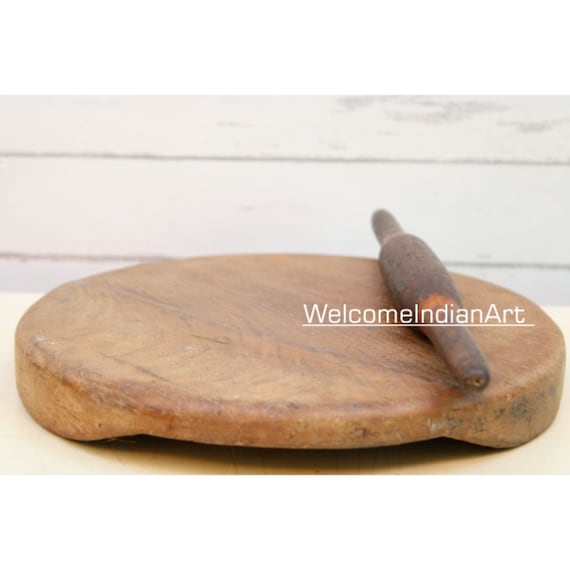The image showcases what looks like an introductory page of a website, designed as a horizontally oriented rectangle. The background displays a light beige surface that resembles wood, featuring darker horizontal lines that suggest wooden boards. The foreground presents a matching light beige countertop, on top of which rests a round cutting board made from darker, smooth-edged wood. Positioned diagonally across the cutting board is a brown rolling pin. Adding to the scene, white text is visible on the right side of the image, reading "Welcome Indian Art," with an underlining white line beneath the text.